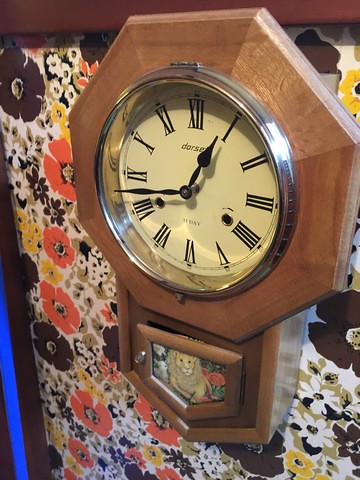This is a photograph of a vintage wall clock taken at a slight angle, with the right side appearing closer than the left. The clock features an octagonal, light golden-colored wooden frame, with a circular clock face enclosed in glass and a silver metal bezel. The face of the clock displays Roman numerals from 1 to 12 and has the name "Dorset" along with the word "Day" inscribed on it. The clock hands, colored black, are positioned just before 1 o'clock and just before 9 o'clock. Below the clock face, there is a small, rectangular door that is slightly ajar. This door has a glass pane and showcases a whimsical painting of a reclining lion amidst red flowers, accompanied by images that might resemble a rabbit and a panda bear. The background of the image is adorned with retro floral wallpaper in hues of black, orange, yellow, and white, characteristic of 1970s decor, and there's a distinct bright blue and black strip visible along the lower left edge.